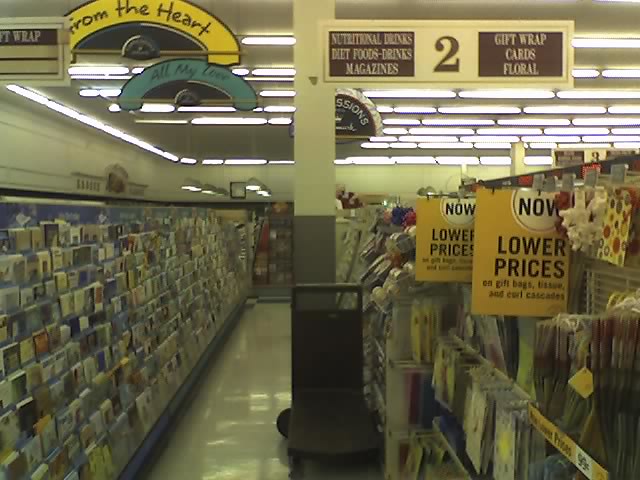In this detailed photograph, we find ourselves situated in the middle of a narrow aisle within a quaint store. The aisle is dedicated to gift wrap and cards, evident from the thematic arrangement of products lining both sides. The shiny off-white tile floor reflects the bright light from the drop ceiling, which features fluorescent lights stretching from left to right. Suspended from the ceiling and attached to a central pillar is a sign indicating "Aisle 2." This pillar is also complemented by a brown trash can placed directly in front of it for convenience.

The sign on the pillar provides a guide to the aisle's contents, listing "nutritional drinks, diet foods, drinks, magazines, and gift wrap, cards, and floral" as its main categories. The left side of the aisle is adorned extensively with rows of colorful gift cards, neatly organized for easy selection. On the opposite side, the right, the upper and lower sections of the shelf showcase an inviting display of gift bags, while the middle section features an array of vibrant wrapping paper rolls extending down the length of the aisle. The composition of the scene delivers a structured yet bustling ambiance common to small, well-stocked retail environments.